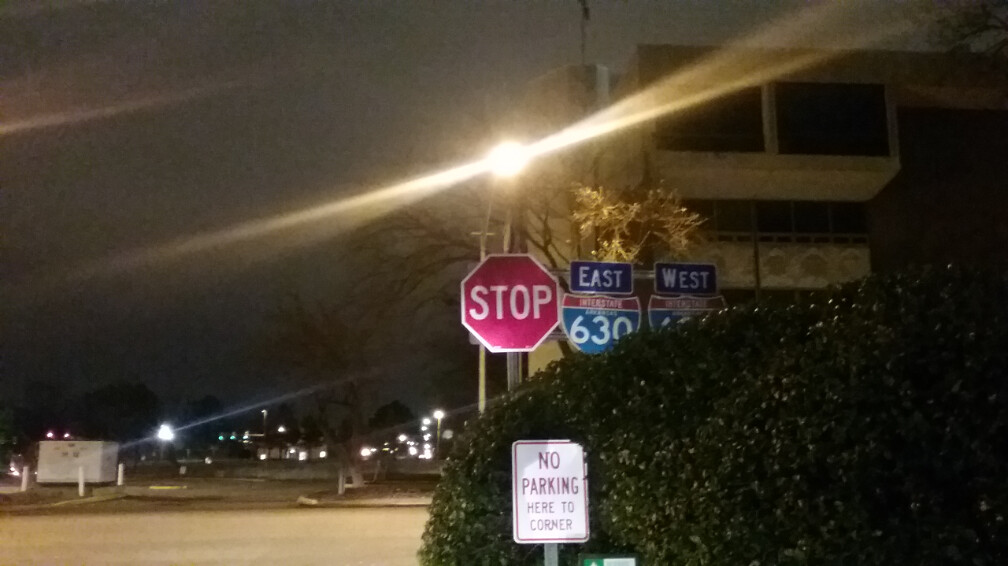The image captures a night scene at a street corner, possibly near a highway intersection. Dominating the center is a red stop sign illuminated by a streetlight directly above it, which casts a radiant glare across the scene. Flanking the stop sign, to the right, are two highway signs: one clearly indicating East Interstate 630 and another partially obscured by a large green bush, likely denoting West Interstate 630. In the lower middle, a white "No Parking Here to Corner" sign with red lettering stands prominently in front of the bush, accompanied by a smaller white and green sign below it. The bottom right corner features this dense bush or hedge. In contrast, the lower left corner reveals faint car lights, hinting at distant vehicles or possibly a nearby parking lot. The upper right of the image is ambiguous, with outlines suggesting either a building or the upper section of an overpass. The overall scene hints at an overpass or freeway exit area, emphasizing the mixed elements of urban infrastructure at night.